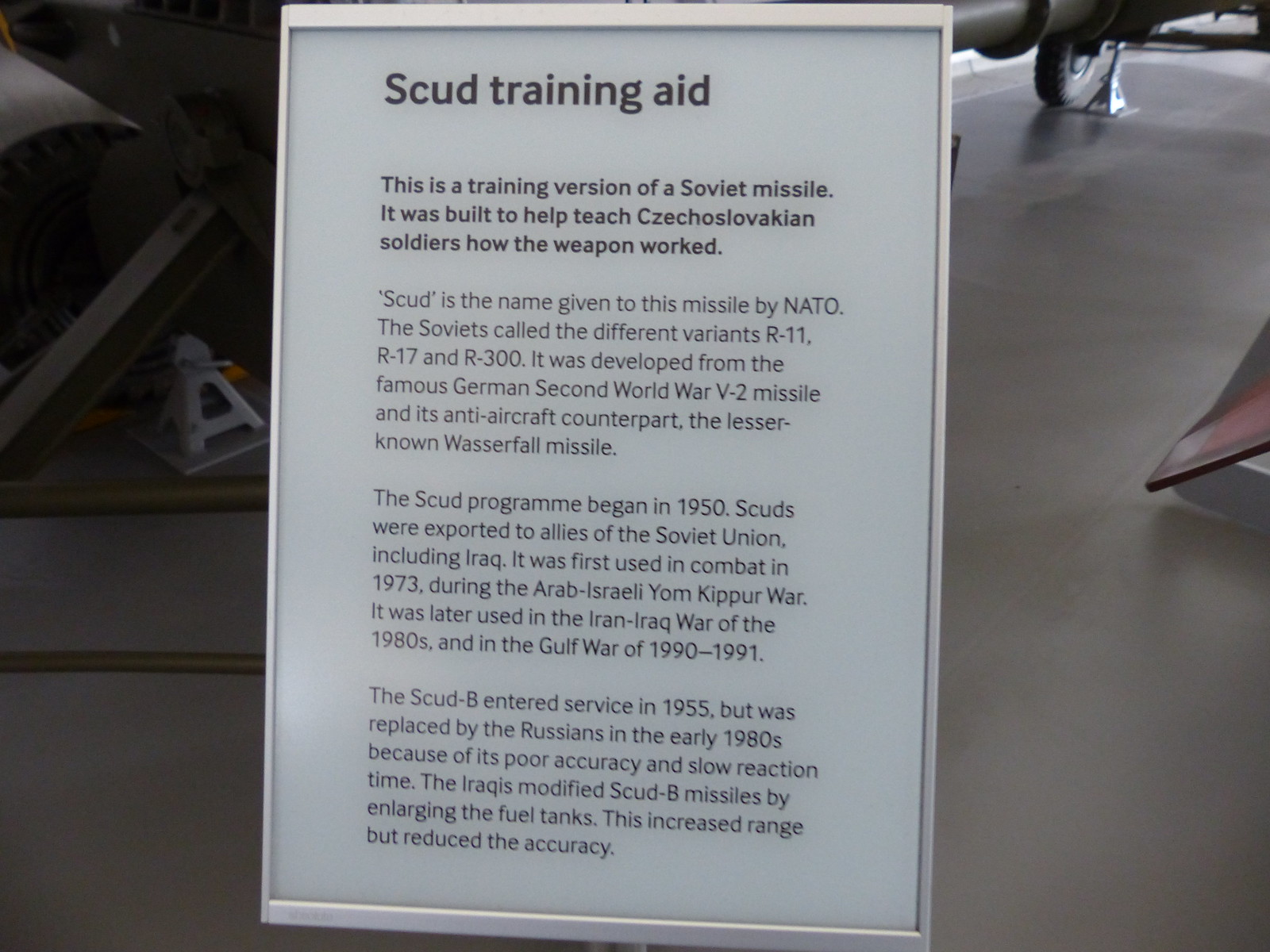The image depicts an informational sign in black and white, situated on what appears to be a piece of machinery or a missile. The sign, framed and centered slightly to the left, reads "Scud Training Aid" and explains that it is a training version of a Soviet missile used to instruct Czechoslovakian soldiers on its operations. This missile, known to NATO as the Scud, has Soviet variants named R-11, R-17, and R-300. Developed from the famous German V-2 missile and its lesser-known anti-aircraft counterpart, the Wasserfall missile, the Scud program began in the 1950s. These missiles were exported to Soviet allies, including Iraq. First used in combat during the Arab-Israeli Yom Kippur War in 1973, Scuds were later utilized in the Iran-Iraq War of the 1980s and the Gulf War between 1990 and 1991. The Scud-B entered service in 1955 but was replaced by the Russians in the early 1980s due to its poor accuracy and slow reaction time. Iraqi modifications to the Scud-B, such as enlarging the fuel tanks, increased its range but further reduced its accuracy. The sign is accompanied by a gray floor, metal parts, and what looks like a wheel, indicating the industrial setting of the display, likely in a museum.